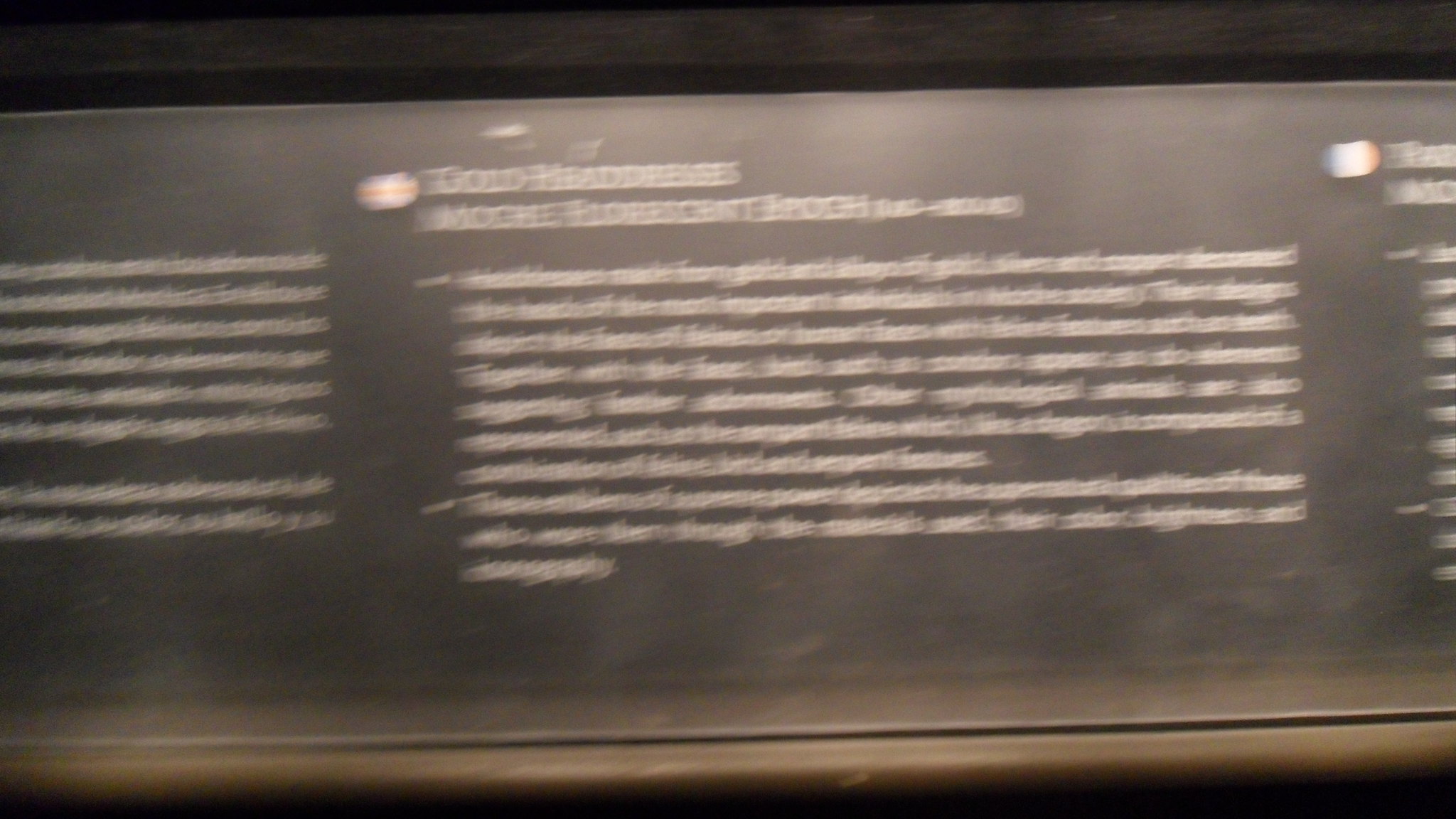This image portrays an extremely blurry, horizontally oriented photograph of a museum plaque or descriptor. The photo's frame is twice as wide as it is tall, featuring dark borders at the top and bottom. At the bottom of the frame, there's a light to dark brown curved object faintly highlighted in white along its front. Above this object is the plaque, which appears to be a dusty dark gray to black in color.

The plaque itself contains significant white text, but due to the blurriness of the image, most of the content is illegible. At the top of the plaque, you can partially read "gold headdresses," "mochi," an unclear word, "epic," and a date, possibly referencing a historical period marked as "something to something A.D." Accompanying these headings, there seems to be a Union Jack flag emblem in a circle to the left, though this detail is also obscured by the poor image quality.

Beneath the headings, the plaque is divided into one and a half large paragraphs of white text rendered in a full-edge format. The text appears to be dense and descriptive, potentially explaining an exhibit or artifact further. However, none of the specific words or sentences within these paragraphs can be discerned due to the significant blurring of the camera. The text layout includes slightly larger font titles that seem to draw attention to particular sections, possibly highlighted by square dots or similar markers.